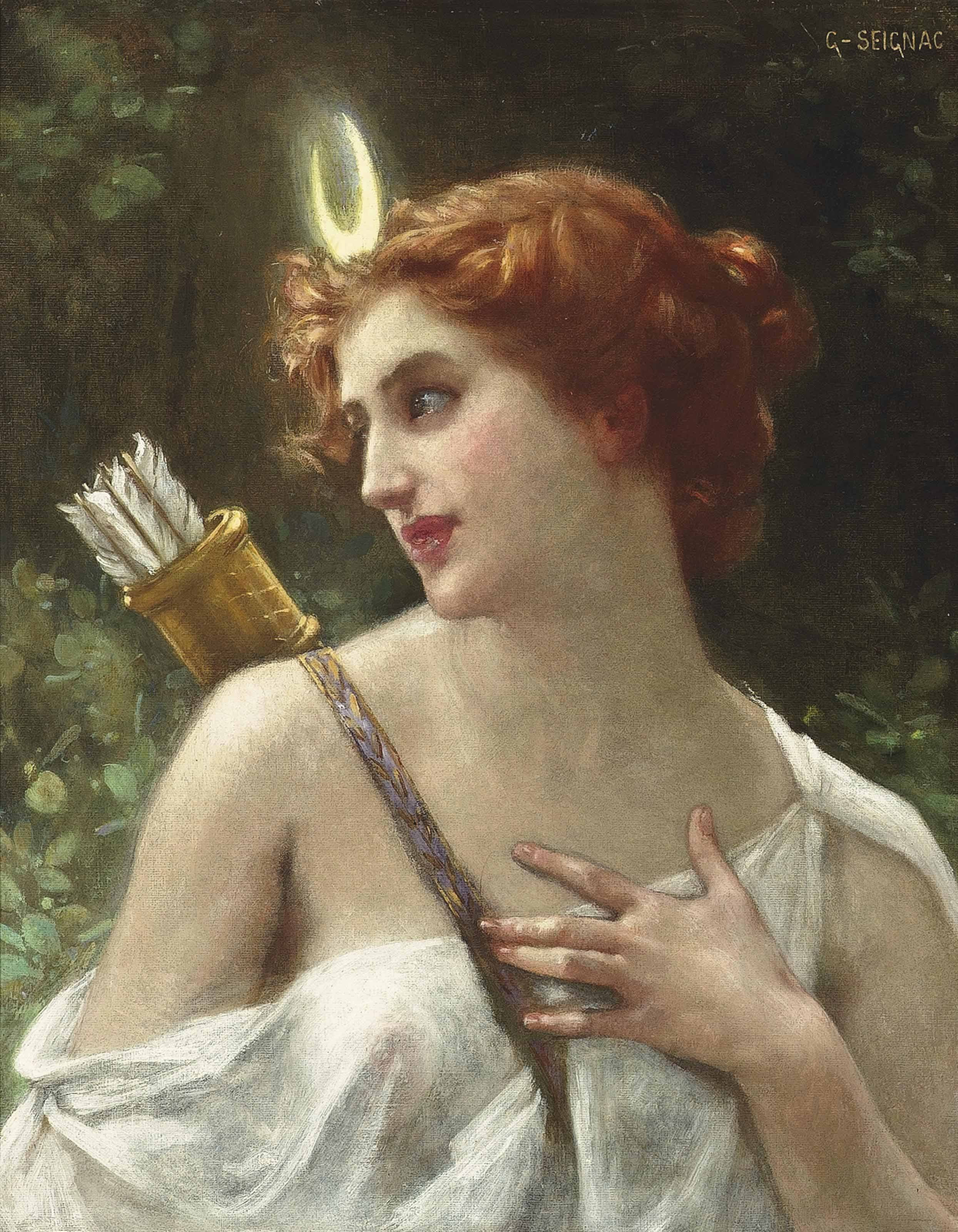This painting is a detailed and beautifully realistic depiction of a woman with a serene and dreamy expression, likely representing an early portrayal of Cupid or a goddess of love. She is adorned in a medieval-style white drape that elegantly covers one shoulder, leaving most of her pale, milky skin and chest exposed. With her hand delicately placed across her chest, she gazes off to the right.

The woman's striking red hair is pulled back and styled away from her face, revealing her bright pink lips. A notable feature is the gold-colored, U-shaped headpiece atop her head, which could be interpreted as a crown or emblem. Over her shoulder, she holds a quiver full of arrows, characterized by a gold body, a brown leather strap, and white feathered arrows peeking out from the top.

The background of the painting is lush with green foliage, accentuating the woman's ethereal presence. The artist's signature, "G-Sagnac," can be seen in the top right corner, further adding to the painting's authentic, historical feel.